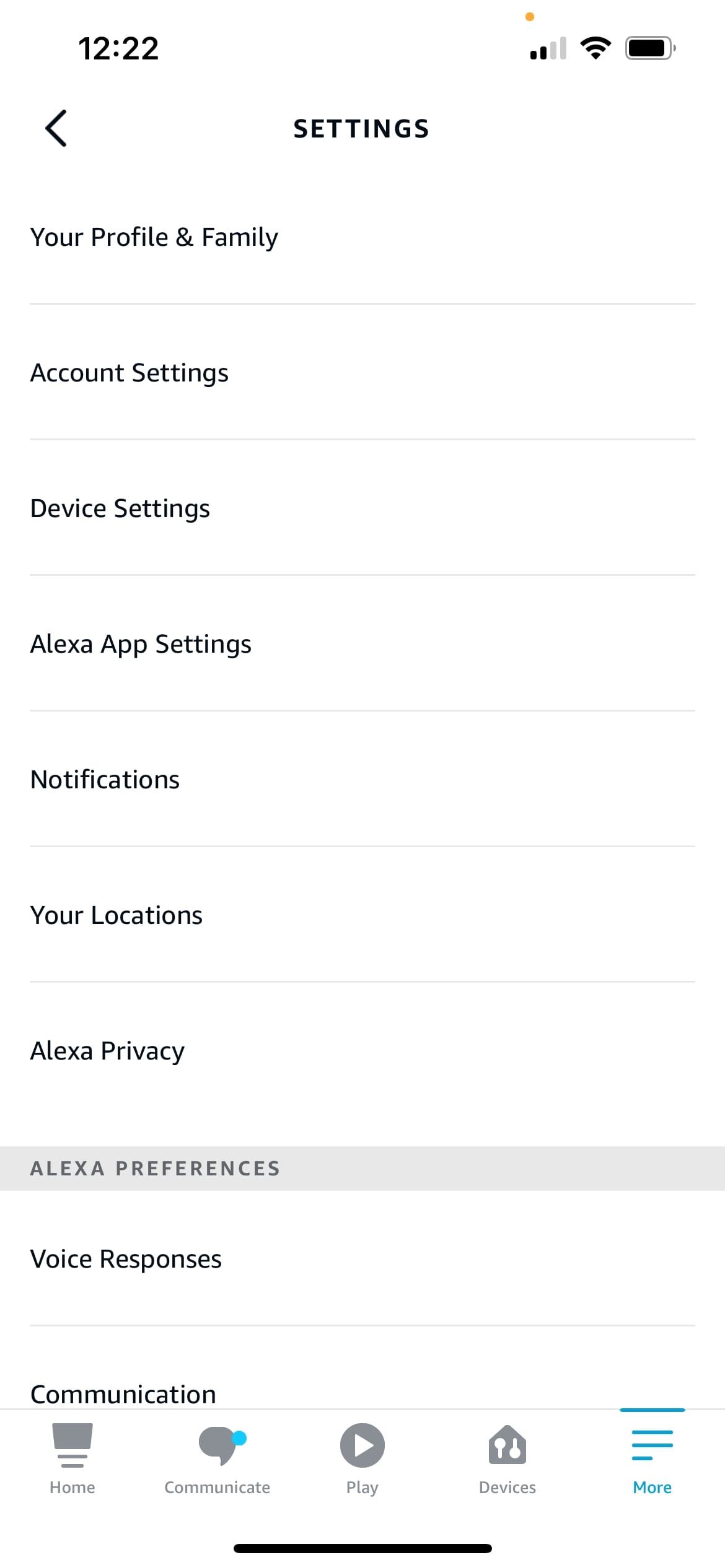The image depicts a smartphone displaying the Alexa app's settings menu. At the top of the screen, the status bar shows a time of 12:22, 2 out of 4 signal bars, a full Wi-Fi indicator, and a battery icon. The settings menu includes several sections under the user's profile and family options. The first section is titled "Account Settings," followed by "Device Settings." 

A distinguished gray bar labeled "Alexa Preferences" is prominently displayed, covering options such as "Voice Responses," "Communication," and "Home." Below this section, the navigation bar includes icons for "Communicate," "Play," "Devices," and "More." The interface uses various shades of blue for highlights and black lines to differentiate between sections, all set against a clean white background. The overall arrangement and visuals suggest a straightforward and user-friendly interface typical of smartphone settings screens.